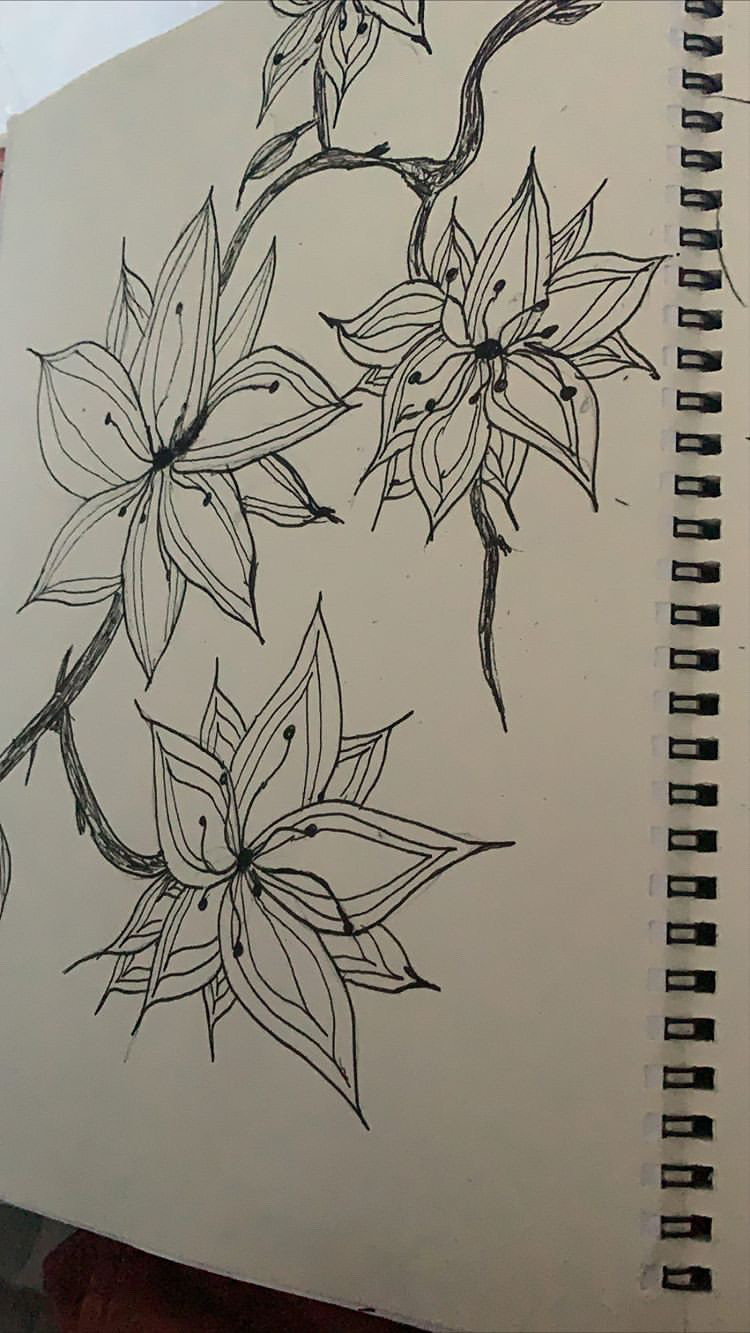This is a detailed black and white line drawing of flowers in a spiral-bound sketchbook. The metal spiral binding is visible on the right-hand side. The off-white page features a complex sketch created with black ink, possibly a marker or Sharpie. Centered around a series of black branches that stretch diagonally from the top right to the bottom left, the drawing depicts four full flowers and a partially visible flower at the top center. Each flower has multiple intricately detailed petals, ranging from nine to twelve, with distinct centers adorned with fine detailing. The pointed petals radiate outward, and several leaves extend from the branches, which appear thorny and bare. The artwork, though monochromatic, suggests the potential vibrancy if colored, enhancing the natural beauty of the depicted flowers.